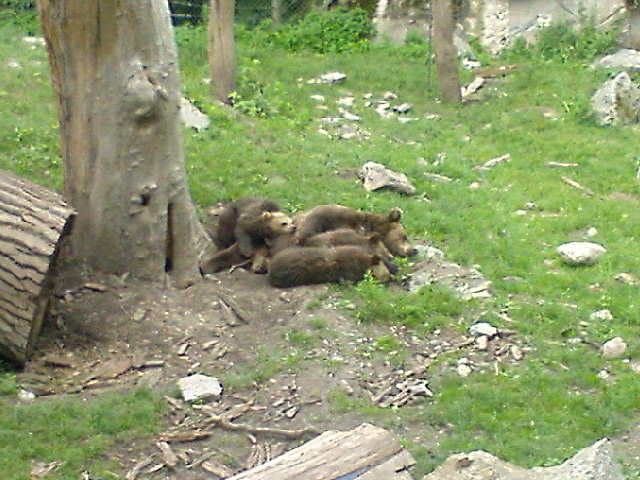The photograph captures a family of brown bears, likely a mother and her cubs, resting in a natural habitat. The scene features four bears with lighter-colored faces, huddled together near a dead tree trunk. The bears are situated in a primarily barren dirt area with some grassy patches and scattered rocks. To the left of the group is a large tumbled-over log next to the thick tree trunk, and partially visible logs are at the bottom of the image. The background, filled with more tree trunks and larger stones, also reveals a chain-link fence, suggesting that the location might be a bear enclosure at a park or zoo. The bears are centrally positioned in the image, appearing to be napping peacefully.